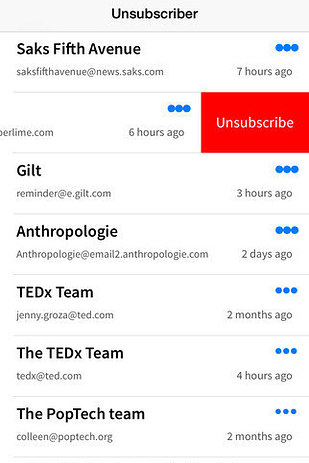The image features a white background with various email notifications, each accompanied by an 'unsubscribe' option. At the top, there is a blue box labeled "Unsubscriber." Below are several email listings:

1. **Saks Fifth Avenue** - The listing includes the sender "Saks Fifth Avenue" from email address "news.saks.com." It shows three blue dots to the right and indicates the email was received seven hours ago.
   
2. **Userlime** - This entry features the sender "Userlime" from "userlime.com" with three blue dots and indicating the email was received six hours ago. A prominent red "Unsubscribe" button is visible here.
   
3. **Guiltreminder** - The listing from "guiltreminder" via "e.guilt.com" shows three blue dots and indicates the email was received three hours ago.
   
4. **Anthropology** - This notification is from "Anthropology" at "email2.anthropology.com," displaying three blue dots and the fact that it was received two days ago.
   
5. **TEDx Team** - Two entries here:
   - The first is from "Jenny Groza" at "jenny.groza@ted.com" received two months ago with three blue dots.
   - The second is from "TEDx Team" at "tedx@ted.com" received four hours ago, marked with three blue dots.
   
6. **Pop Tech Team** - The final listing is from "Pop Tech Team" with the sender email "colleen@poptech.org," received two months ago, accompanied by three blue dots.

This collage of notifications provides insight into various promotional and informational emails received over time, each with an option to unsubscribe.